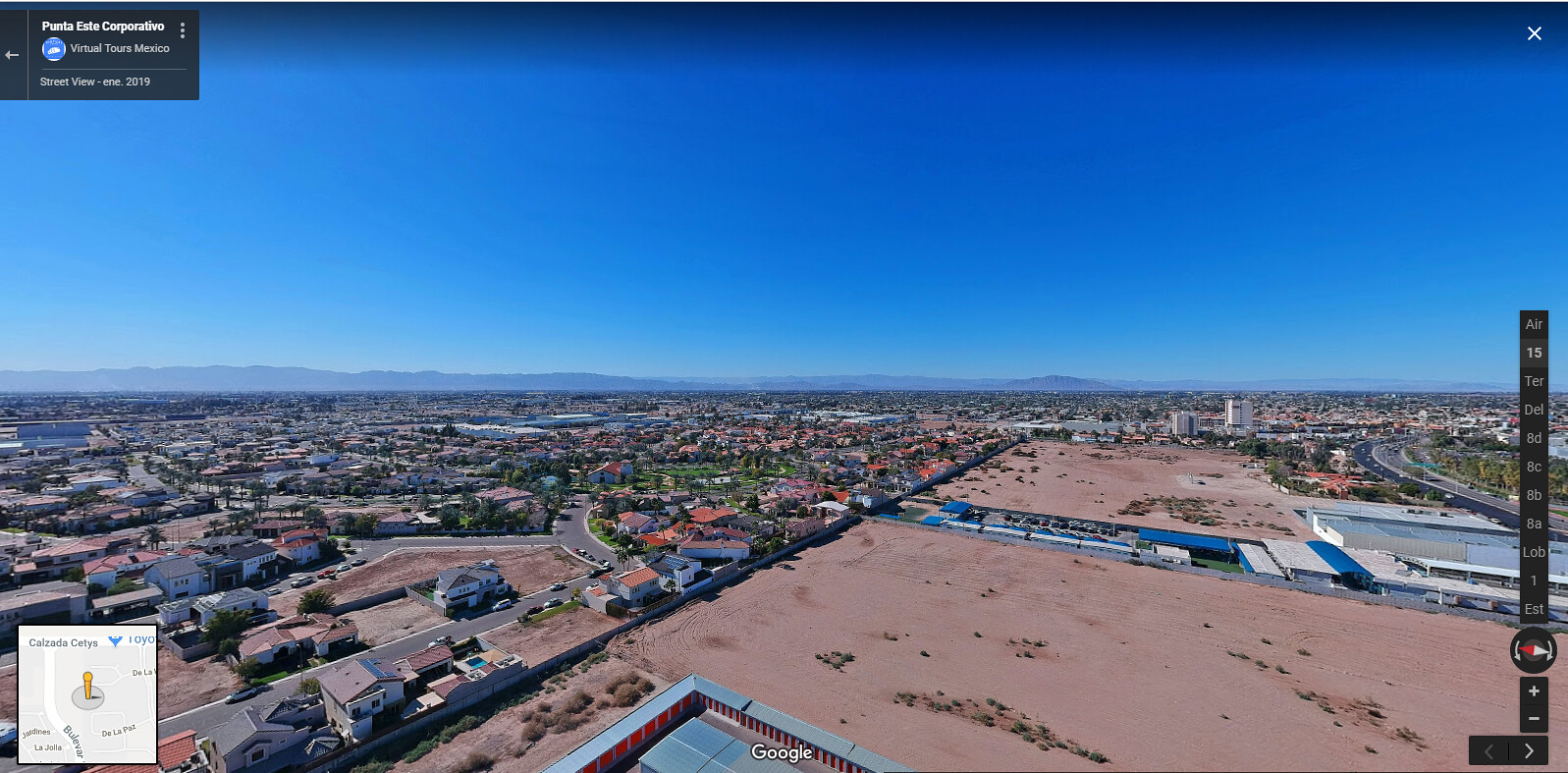A high-resolution satellite image from Google Earth showcases the scenic landscape of Punta Esta Cooperative in Mexico, captured in 2019. The image features a stunning blue sky set against a backdrop of majestic mountains, with a mix of developed and undeveloped areas below. To the center and right are neatly arranged housing developments that give way to a more sandy, untouched terrain. 

In the top left corner, the label reads "Punta Esta Cooperative, Virtual Tours Mexico, Street View from 2019," providing context to the scene. The bottom left corner indicates map coordinates, pinpointing the location near Budweiser or Budford Highway and Calzada Seta. 

On the right side of the image, the navigation options are displayed, including a compass for orientation. This section features a vertical column of navigation commands, listed as AIR, 15, TER, DEL, 8D, 8C, 8B, 8A, LOB, and EST, presumably offering various viewing or traversal options. Beneath this column, plus and minus buttons allow users to zoom in or out.

Overall, the view is zoomed out, providing an aerial perspective that showcases both the vastness and the intricate details of the landscape below. This image is part of a virtual tour, offering a high vantage point that encapsulates the natural and developed beauty of Punta Esta Cooperative.